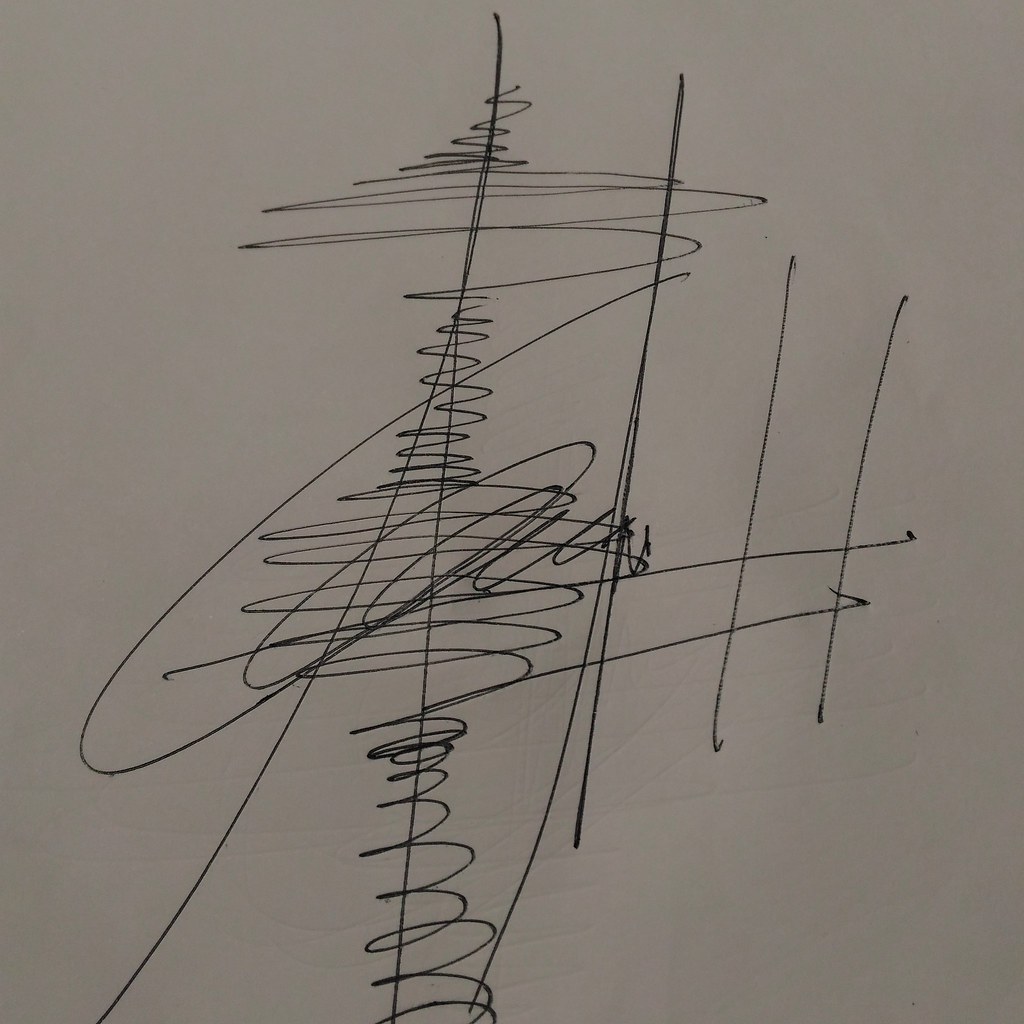The image features a computer-generated artwork set against a uniform grey-brown background, devoid of any other colors or textures. The composition predominantly comprises an array of black pen lines. Beginning at the bottom center of the image, there is a corkscrew-shaped spring resembling a car suspension component. This spring coils vertically upwards, anchored by a straight vertical line that extends uninterrupted to the top edge of the image. 

Above the spring section, there is a transitional gap, followed by an intricate network of circles and squiggles that perpetuate the design's vertical flow towards the top. In addition to the main vertical line, there are three other prominent vertical lines situated to its right. These lines are intermittently crossed by two horizontal lines. Additionally, a slanted line ascends from the bottom left, sweeping upwards and merging with the main vertical line near the top of the image.

The artwork's intricate play of straight and coiled elements, combined with the detailed overlay of squiggles, creates a visually compelling pattern that suggests a computer's precise hand in its creation.